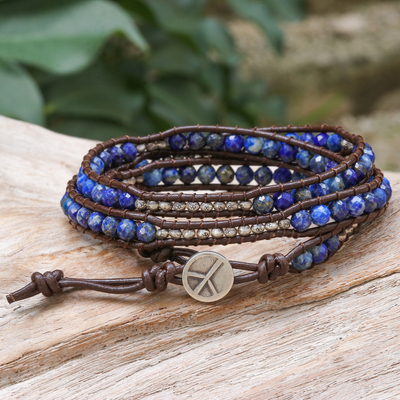This image captures a prominently detailed leather bracelet, which appears to be of a multi-wrap style, set against a natural backdrop. The bracelet, made of dark brown leather, features intricate beading with numerous blue and silver beads interspersed with knots. The blue beads are a vibrant, deep shade with white marbling, and some also display subtle hints of yellow, giving them a splotchy, multi-colored appearance. Among these, smaller pearl-colored and shiny silver beads add to the intricate design.

The bracelet showcases two distinct tracks of beading and knots, with a notable centerpiece—a large silver pendant featuring a peace symbol, acting as a clasp. The entire piece is coiled and laid out on a wooden surface, framed by green leaves, hinting at an outdoor setting. The photograph is taken from a direct, slightly crouched angle, emphasizing the bracelet's detailed craftsmanship and the contrasting textures of leather, beads, and natural elements.